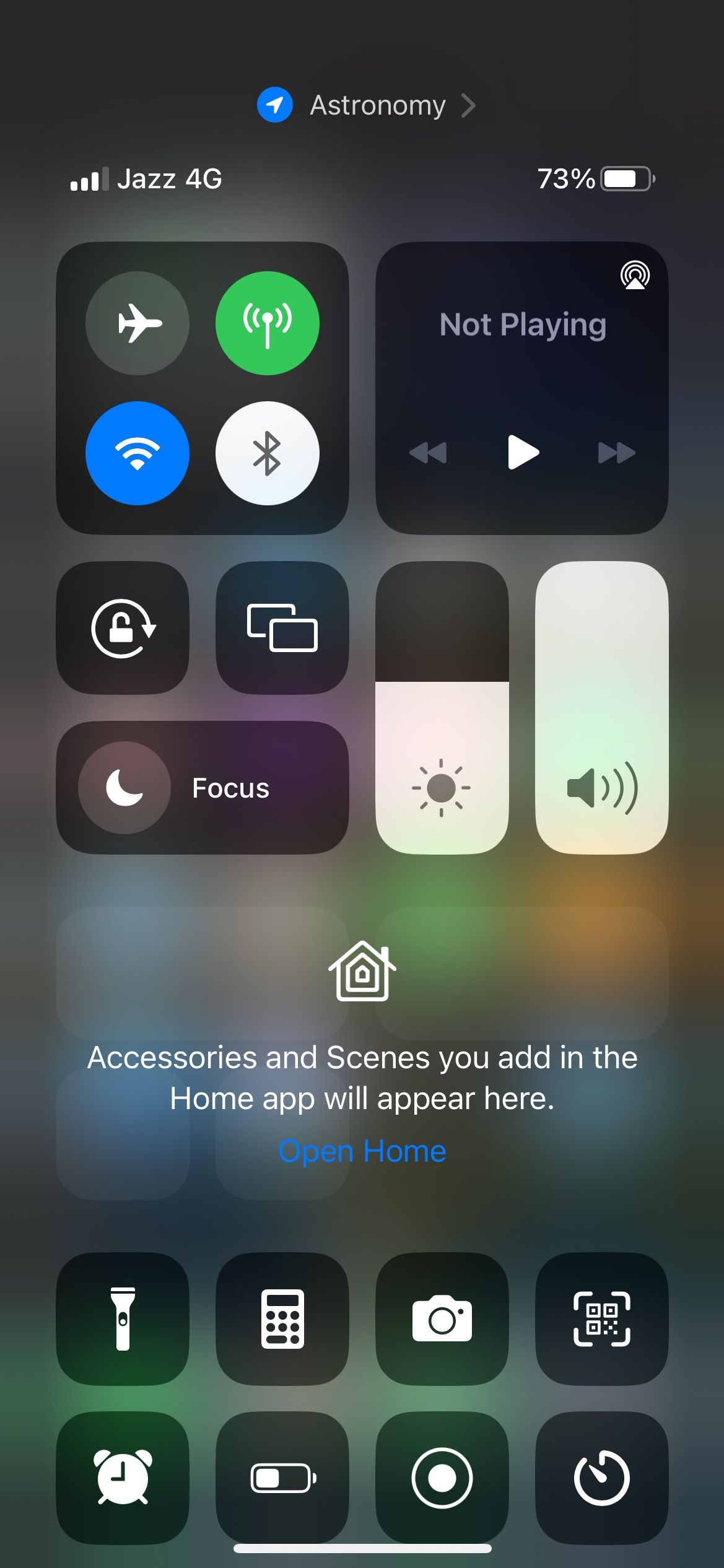The image depicts a detailed view of a smartphone control center interface. In the top right corner, there is a blue circle icon for location services, labeled "Astronomy," displaying a status of 73%. On the top left, the cellular network status shows "Jazz 4G" with three out of four bars filled, indicating signal strength. Airplane mode is enabled, represented by its icon. A green circle icon indicates active radio signals, such as cell data. The Wi-Fi button is illuminated in blue, signaling that Wi-Fi is active, while the Bluetooth button is white, indicating it is inactive or disconnected.

Further to the right, music playback controls are shown, including a "Not Playing" status, a play button, and fast forward and rewind buttons. There is also a lock icon for screen rotation control and a screen mirroring button. The brightness control appears as a gray slider.

Adjacent to these features, a gray speaker icon and a grayscale focus mode icon are displayed. A white moon icon signifies that Do Not Disturb mode is active. Next, there is a home section displaying white text stating, "Accessories and scenes you add in the Home app will appear here. Open Home." 

Additional controls at the bottom include a flashlight with a white symbol, a calculator button, a camera button, a QR code reader, and a clock icon. The battery icon shows it is halfway charged, accompanied by a circular tape symbol and an additional clock icon.